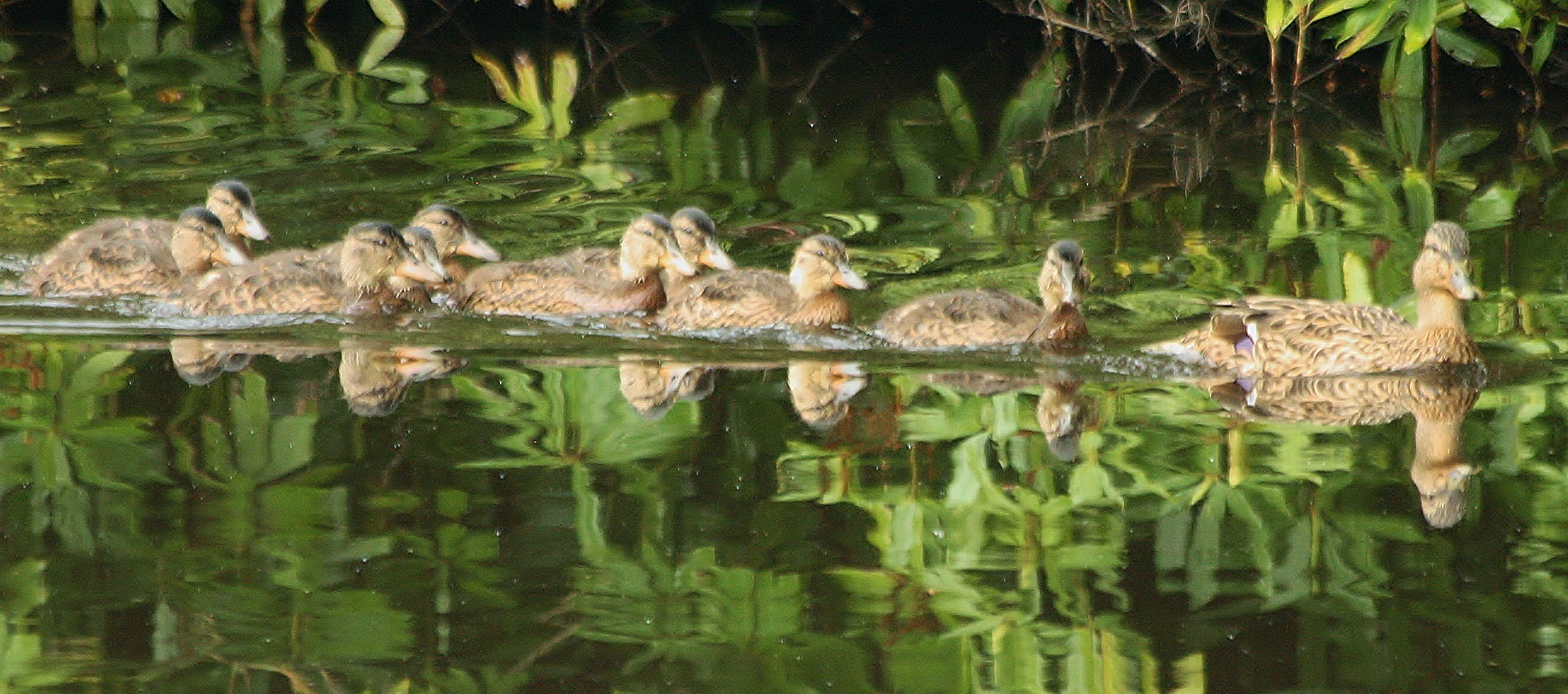This landscape-style photograph captures a serene scene of nine ducks swimming in a pond, moving in a line from left to right. The water is a calm green, highly reflective, mirroring the pale green leaves from trees and bushes above. The ducks, likely a mother followed by her juveniles, share a distinctive coloration: their heads are slightly darker with a black strip down the center, brown on the sides, and their necks. Their bodies are primarily brown with black specks and a pattern of black and white on their tails. The largest duck, positioned centrally with its head turned towards the camera, leads the group. The second and third ducks also glance toward the camera, while the others look forward. In the water beneath them, their yellowish-gold bodies and dark gray beaks are clearly reflected. The pond's surface is mostly undisturbed save for the gentle ripples created by the ducks' movement, and the water extends from the bottom up to near the top of the image, where a few leaves and sticks intrude slightly from the upper corners.